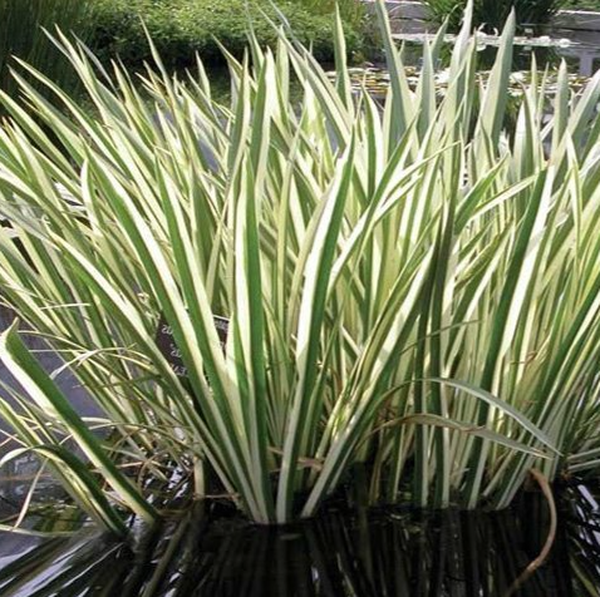A detailed, close-up photograph showcases a vibrant clump of two-tone, blade-like leaves, approximately half green and half off-white, sprouting in abundance from the base. These reed-like plants are situated at the edge of a pond, partially obscuring the brownish water and floating debris behind them. A faint reflection in the water adds to the serene outdoor setting. In the background, greenery and shrubbery intertwine, alongside what appears to be a stone ledge, enhancing the natural ambiance. A small sign featuring white text is subtly positioned slightly left of center in the image, adding a point of interest amid the lush foliage.